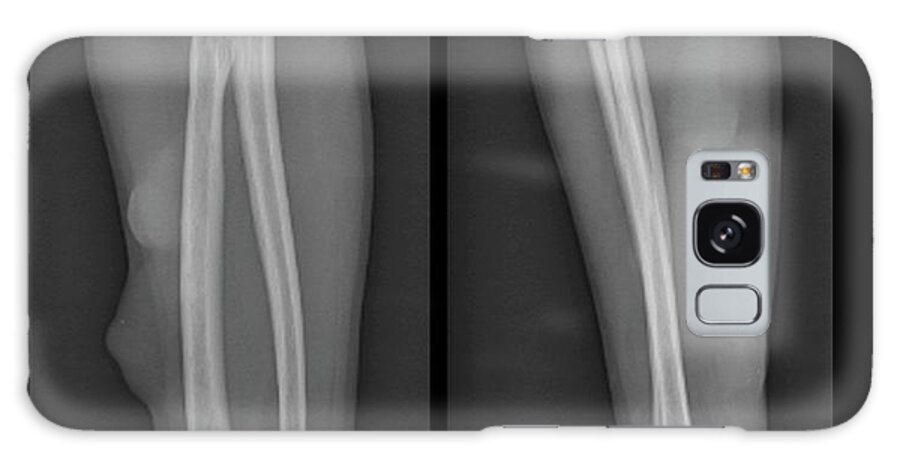The image features a smartphone placed on its side, showcasing a distinctive phone case. The case is predominantly in black and white and has an intricate pattern resembling x-rays, giving it a photorealistic feel despite being likely an illustration. The phone case design splits down the middle with a black bar, creating two mirrored sections. On the left side of the case, the x-ray reveals what appear to be two bones within muscle-like structures, while the right side shows a similar singular bone portrayal. The right side of the phone displays the camera setup, which includes a prominent black lens centrally located, smaller lenses above it, and a white-colored lens near the bottom. The case is designed with little notches along the top, bottom, and left side and features rounded corners. The overall palette consists of dark gray, black, and varying shades of gray and white, adding to the x-ray aesthetic that gives the case its unique visual appeal.